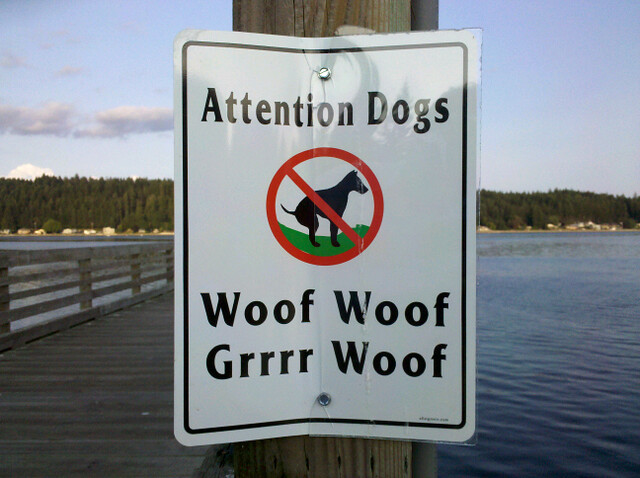The image captures an early dawn scene with the sky transitioning from soft purple to pink hues. At the entrance of a wooden pier that stretches out over a serene lake, there's a large wooden post with a laminated white sign affixed to it. The sign, outlined in black, prominently displays the text "ATTENTION DOGS!" followed by "woof woof, grr woof." In the center of the sign, a graphic depicts a black silhouette of a dog squatting on grass, encircled by a red circle with a diagonal slash through it, indicating a no-dogs-allowed policy. The pier itself is constructed with wooden planks and railings, extending over the tranquil water which reflects the morning light. Across the lake, the shoreline is dotted with large evergreen trees and sandy beaches, adding to the picturesque quality of the scene.